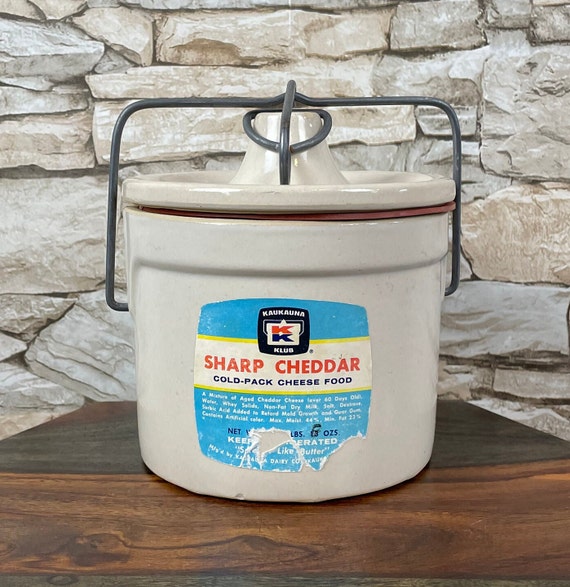The photograph features a large, off-white porcelain crock situated on a dark wooden surface, against a background of an off-white, semi-rectangular stone wall with light brown accents. The crock is equipped with a distinctive metal locking mechanism on the top, providing a secure seal. The centerpiece of the crock is a prominently displayed, albeit weathered and partially torn, blue and white label that reads "Sharp Cheddar" in bold red letters, below which, in black text, it states "Cold Pack Cheese Food." The label indicates the product comes from the Kalakuana Club, though some of the finer details are obscured due to damage on the label. Despite being labeled "cheese food," suggesting it is not real cheese, the packaging conveys an impression of quality. The reflective, shiny surface of the crock, possibly enhanced by paint, contributes to its convincing, premium appearance.